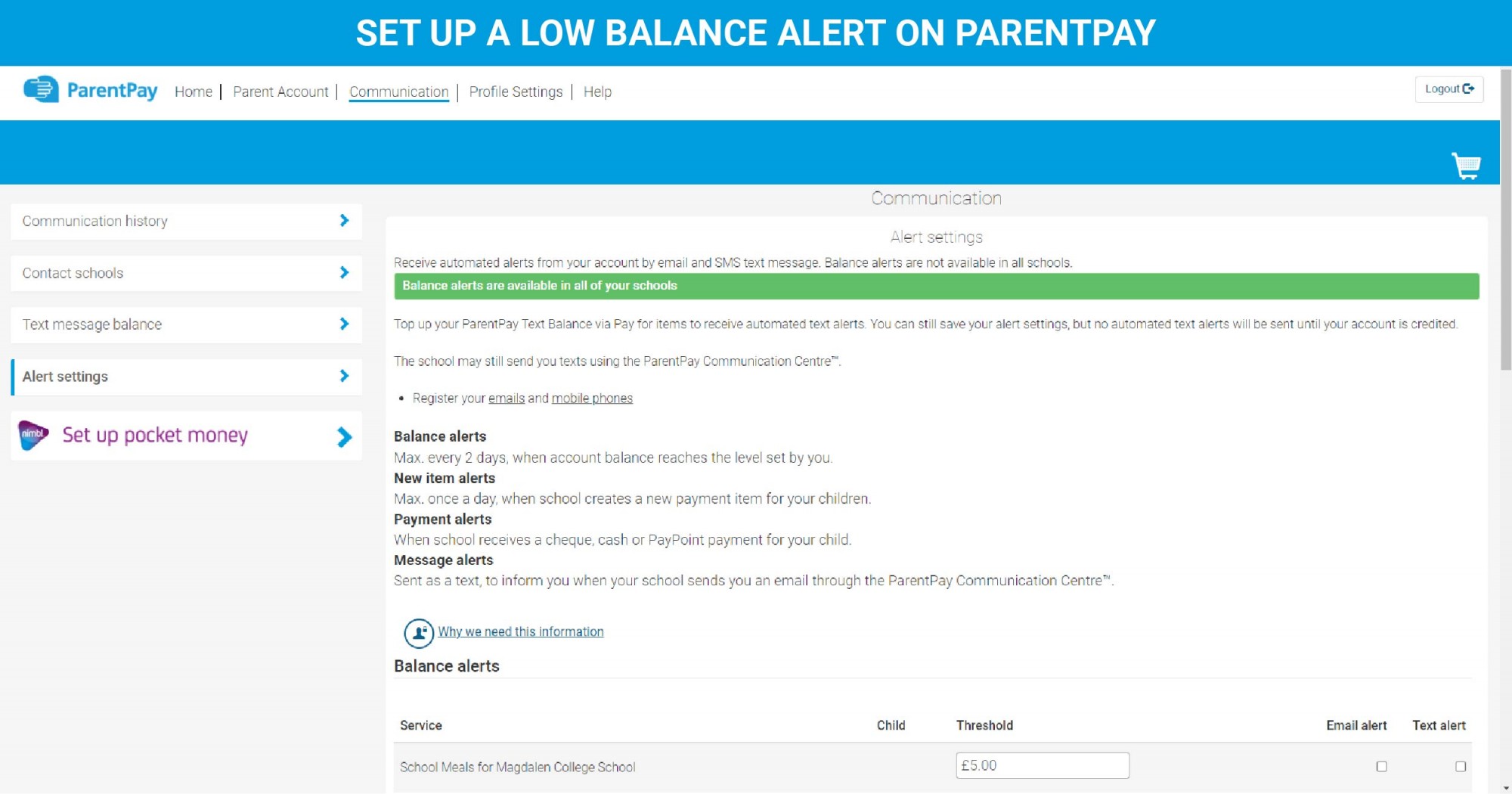Screenshot Description:

The user interface of the ParentPay platform is displayed on the screen, featuring a blue navigation bar at the top and several menus labeled "Parent Pay Home," "Parent Account," "Communication," "Profile Settings," "Help," and "Logout." Below the blue bar, the interface provides access to the communication history, contact options for the school, text message balance, alert settings, and the setup for pocket money. The purple text highlights the "Communication" and "Alert Settings" sections.

The "Alert Settings" section elaborates on how to receive automated alerts from the ParentPay account, available through email or SMS. A notice mentions that alert availability may vary by school. The screen indicates that balance alerts are enabled for all schools associated with the account.

Users are prompted to top-up their ParentPay text balance via the "Pay for Items" option to continue receiving automated text alerts. Although alert settings can be saved, text alerts won't be sent until the account balance is recredited. Schools, however, may still send texts using ParentPay communication tools.

Various alert types are described, including:
- Balance alerts: Triggered based on the account balance threshold set by users.
- New item alerts: Notify parents when new payment items are created by the school.
- Payment alerts: Inform parents when the school receives a check, cash, or PayPoint payment for their child.
- Message alerts: Sent as texts to notify parents when the school sends an email via ParentPay.

Examples illustrate specific alerts for Magdalene College School, including a balance alert threshold set at £5, with both email and text alerts currently unchecked.

A scroll bar on the right side of the screen suggests more content is available to view.